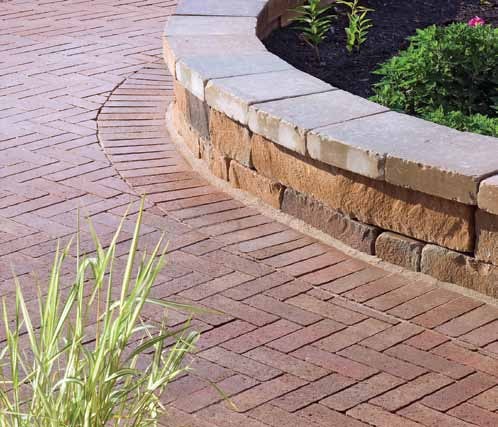The photo captures an outdoor scene featuring a curved concrete walkway made of red bricks, which form a serpentine pattern. Adjacent to the path on the upper right side, there is a small, three-layer high stone wall constructed from gray, reddish, and black stones. This wall frames a raised flower bed with dark, fresh mulch. Within the mulch, several green plants and bushes are visible, along with a solitary blooming pink flower. The pathway closely follows the curve of the stone wall, where the bricks are meticulously laid side by side, transitioning into various orientations further along the walkway. On the very bottom left of the image, patches of green, spiky grass can be seen. This detailed scene encapsulates a harmoniously designed and lush garden area, partially enclosed by the stone wall and flanked by the winding brick path.